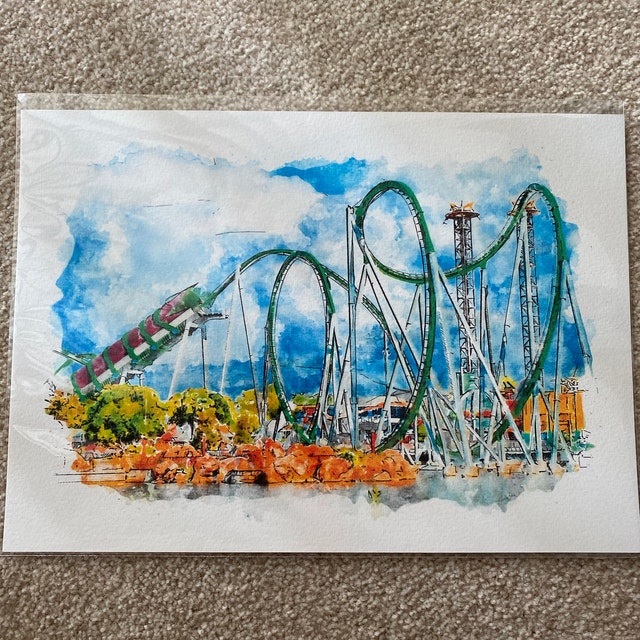A detailed watercolor and ink painting captures a vibrant roller coaster against a blue sky scattered with white clouds. The roller coaster's green tubular structure performs several loop-the-loops, supported by white metal pipes and towers. The coaster car, adorned in purple, white, and green, begins its ascent on the left side of the track. Below the coaster, a mix of lush green trees and striking orange rocks adds to the scenic landscape. The print, encased in a clear cellophane bag, lies on a beige carpet, highlighting the artwork's vivid details and dynamic composition.